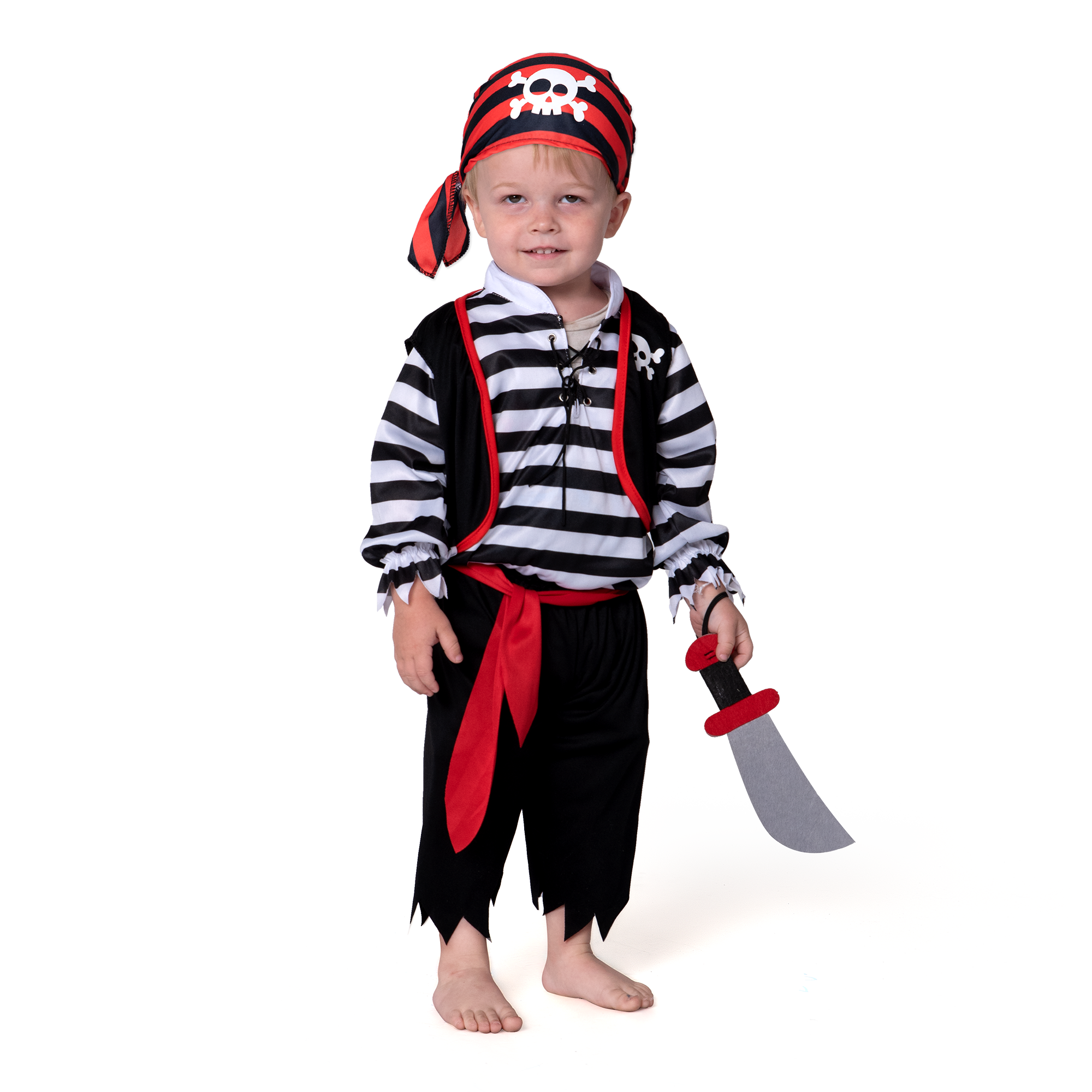This photograph showcases a young blonde boy, around three to five years old, clad in an elaborate pirate costume, likely aimed at promoting sales of the outfit. He stands barefoot against a completely white backdrop, gazing directly at the camera. The boy's attire includes black pants with ragged edges, tied at the waist with a red sash. He sports a horizontally striped black-and-white top, layered under a black and red bolero jacket emblazoned with a white skull emblem, matching the skull on his red and black striped bandana. In his left hand, he brandishes a plastic red, black, and silver saber, completing his pirate ensemble.